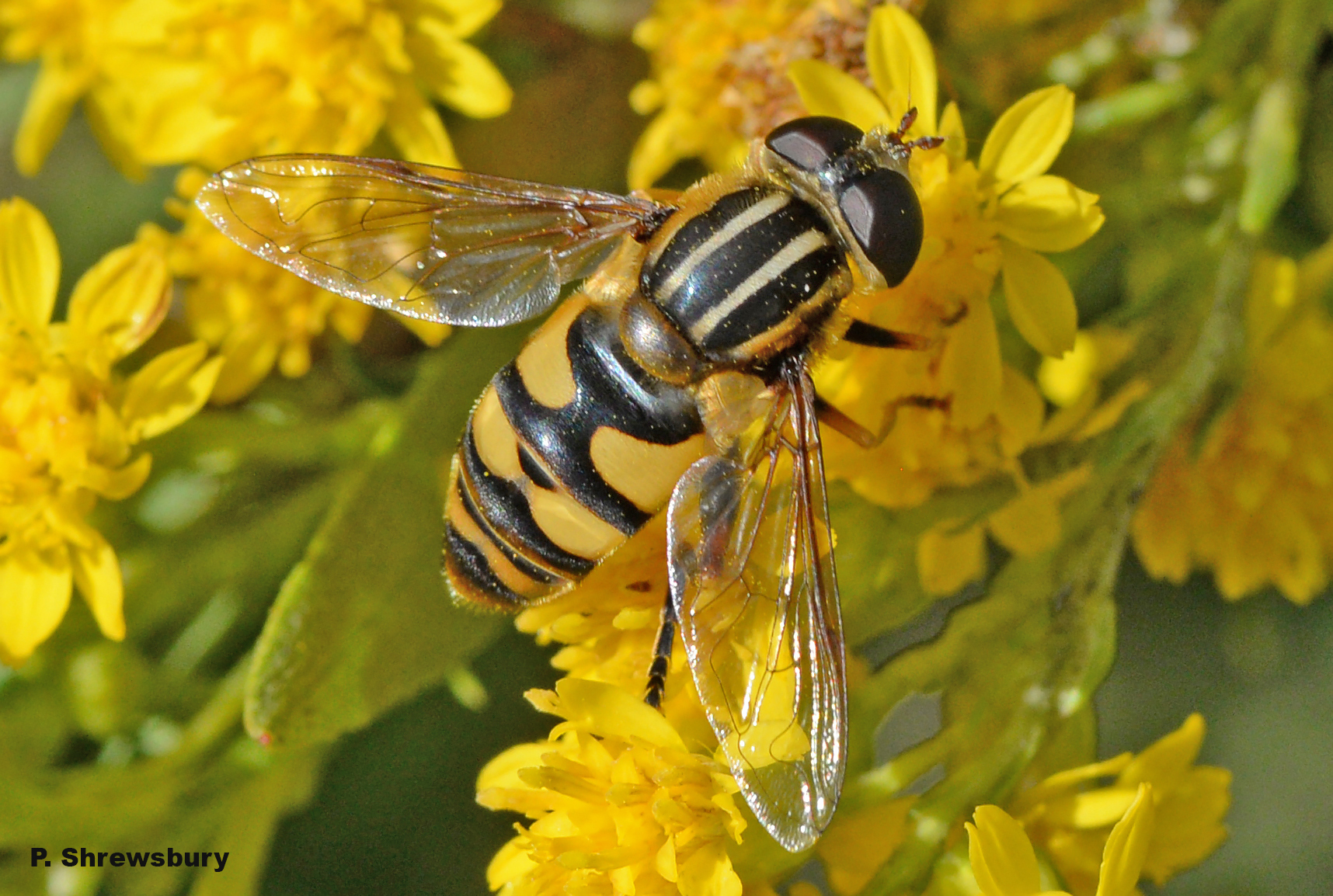This detailed close-up photograph captures a bee resting on a bright yellow flower. The bee, prominently centered in the horizontal image, is nestled among the flower's numerous small petals and yellow center, preparing to pollinate. Surrounding the bee, more yellow flowers and green leaves create a vibrant, blurred backdrop that emphasizes the outdoor, daytime setting in nature.

The bee's striking appearance features large black eyes and two small brown antennas on its head. Its upper body is dark, contrasted by its elongate, pointy abdomen adorned with yellow and black stripes and yellow fuzz towards the tail. Two translucent wings with intricate brown vein patterns fan out slightly from its back, while its brown legs cling to the flower. This detailed image highlights the intricate beauty of a bee in its natural environment.